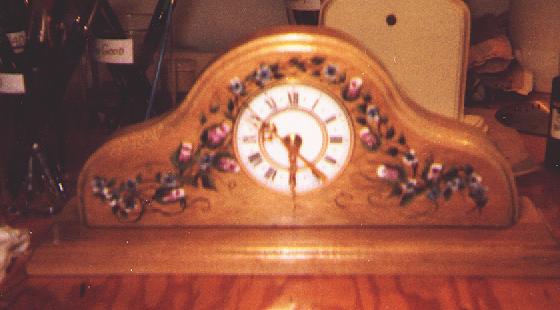A wooden mantelpiece clock is elegantly displayed on a matching light brown rectangular wooden base. The clock features a polished light brown finish. The structure of the clock is characterized by a central dome flanked by two smaller curved shoulders. The clock face, encased in the central dome, is adorned with delicate pink rosebud paintings along the sides and top, complemented by dark green foliage. The face itself is white, with ornate gold Roman numerals marking the hours. Fine gold hands indicate the time as approximately 5:51. Behind the clock on the left side, containers filled with paintbrushes add an artistic touch to the scene. The entire setup rests on a light brown wooden table.